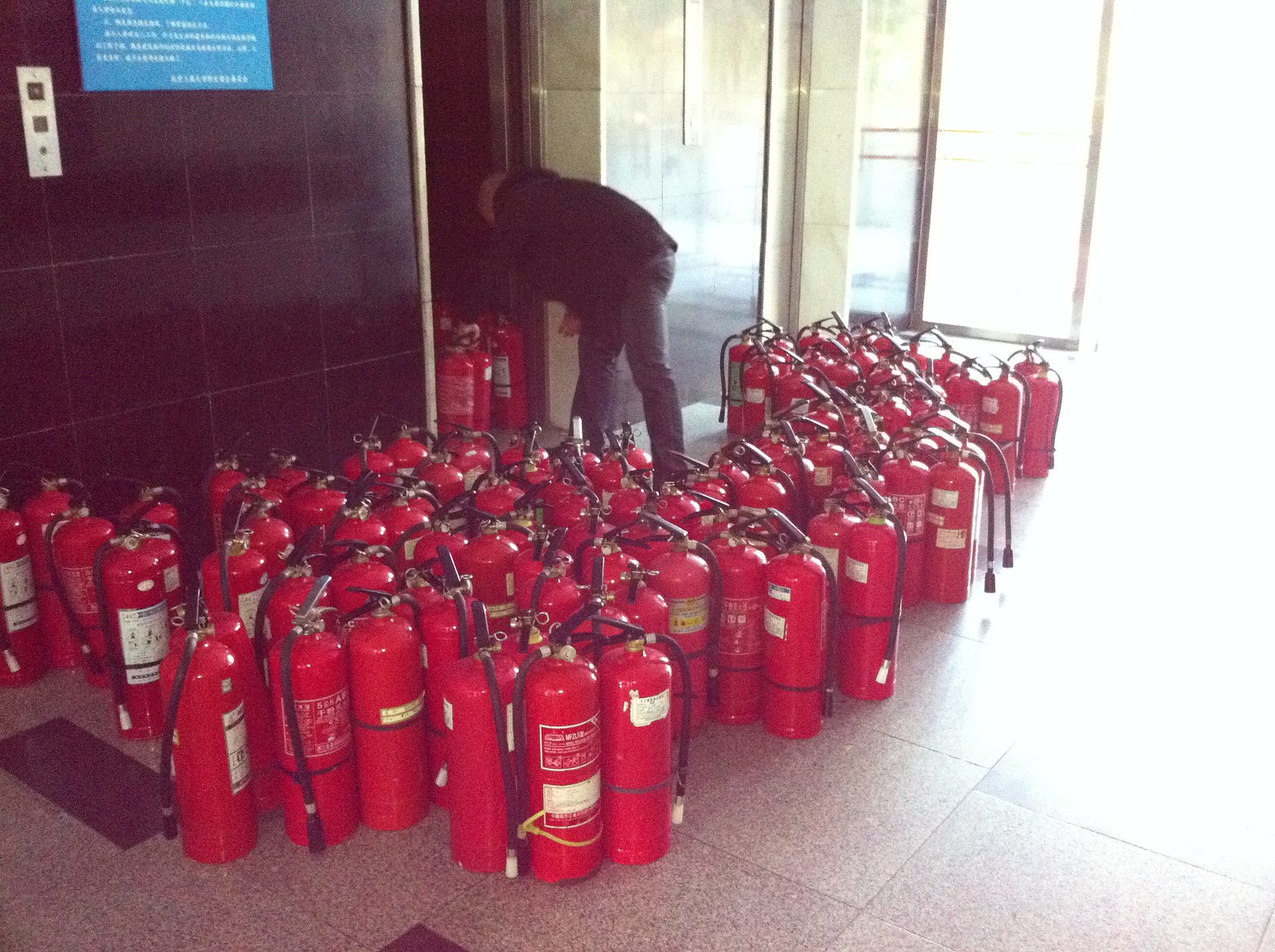A man wearing a black jacket and blue jeans stands in the lobby of a building, surrounded by an extensive array of red fire extinguishers spread across a gray and white speckled tile floor. In front of him is an open elevator door from which he is retrieving more fire extinguishers, adding to the numerous ones already sprawled around him. The scene shows a black wall with elevator call buttons featuring up and down arrows, and to the far right, there are large glass doors letting in a lot of sunlight, indicating an exterior entrance. The man appears to be involved in checking, maintaining, or transporting the fire extinguishers within this large building complex.